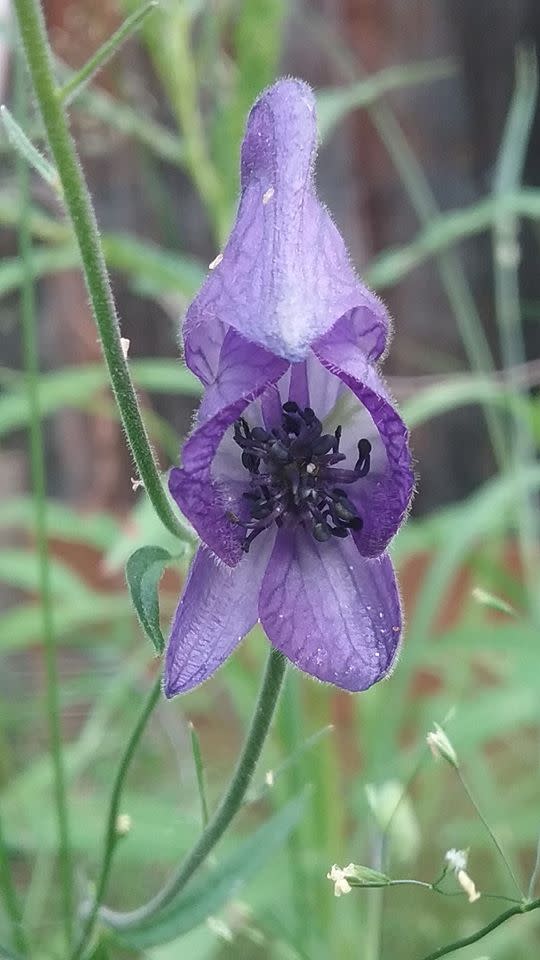This vibrant, close-up color photograph, taken outdoors during the daytime, focuses on a striking purple flower just starting to bloom. The flower, partially open, reveals its blackish-purple seeds nestled inside. The petals, numbered between five and eight, showcase a deep, dark purple hue accented by fine white veins and a hint of white at their edges. These petals are arranged in distinct layers, giving the bloom a multi-layered appearance with very fine fuzz covering their surface. 

The flower is borne on a hairy green stem, extending upward amidst a backdrop of softly focused stems and narrow leaves, creating a well-lit, colorful garden scene. The detailed texture of the petals and the fine hairs on the stem are clearly visible, enhancing the delicate beauty of the flower. Accompanying this main bloom are a few buds on the same plant, yet to open but promising similar purple flowers. Additionally, tiny white flowers from a nearby plant appear in the bottom right corner of the image, contributing to the lush greenery that frames the main subject. The bright, natural light illuminates the entire scene, highlighting the intricate details and vivid colors of the flower and its surroundings.